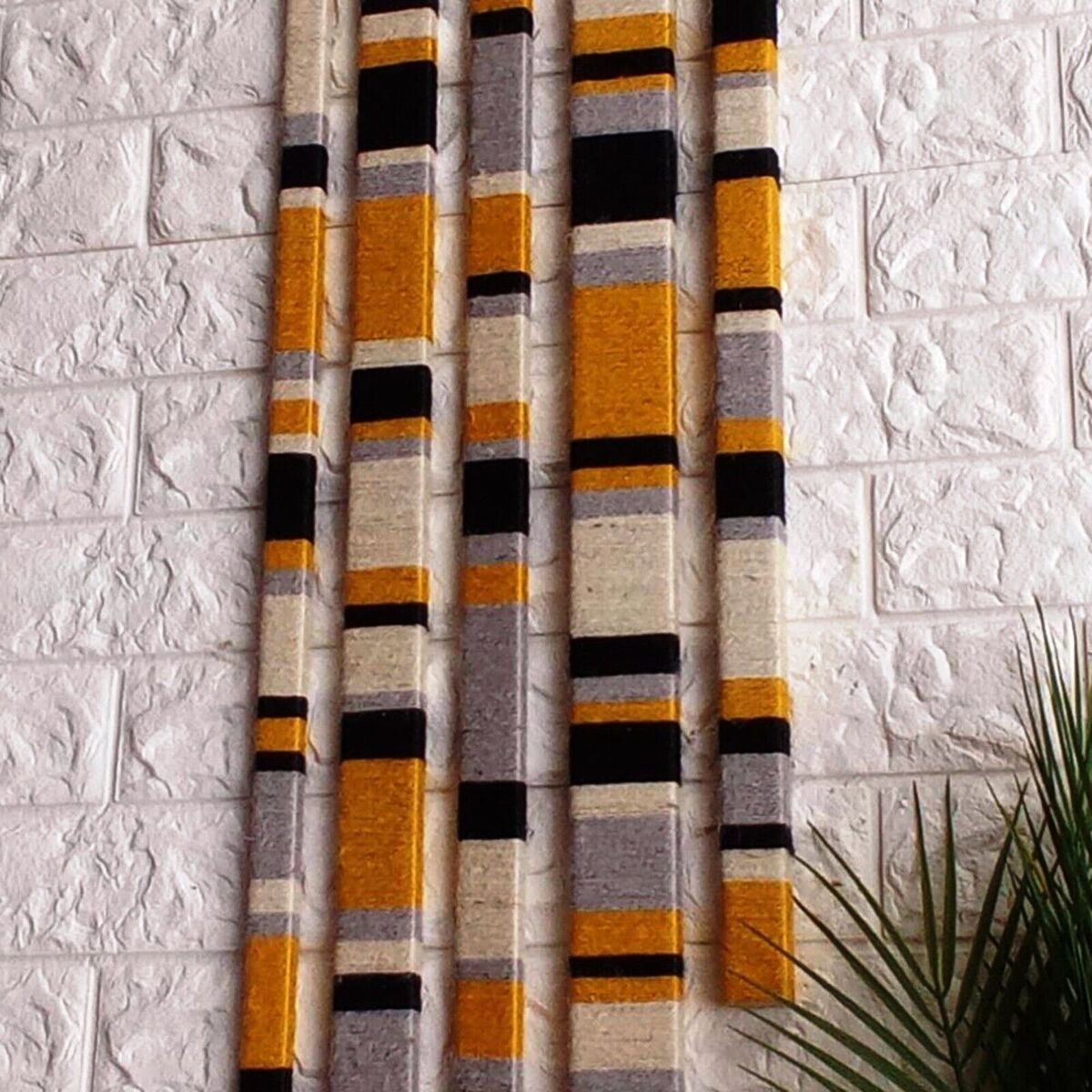The photograph depicts a textured white concrete wall sectioned to resemble bricks. In the bottom right corner, a cluster of green palm fronds stretches upward. Dominating the center of the image are five vertically hanging, post-like objects that vary in width and length. Each object is wrapped in bands of colorful yarn, featuring hues of cream, gray, black, and orange. These rows, described as long boards or sculptural pieces, create a striking decorative pattern against the wall. The objects appear to be connected by thin, void-like threads, adding an intricate detail to the visual arrangement.